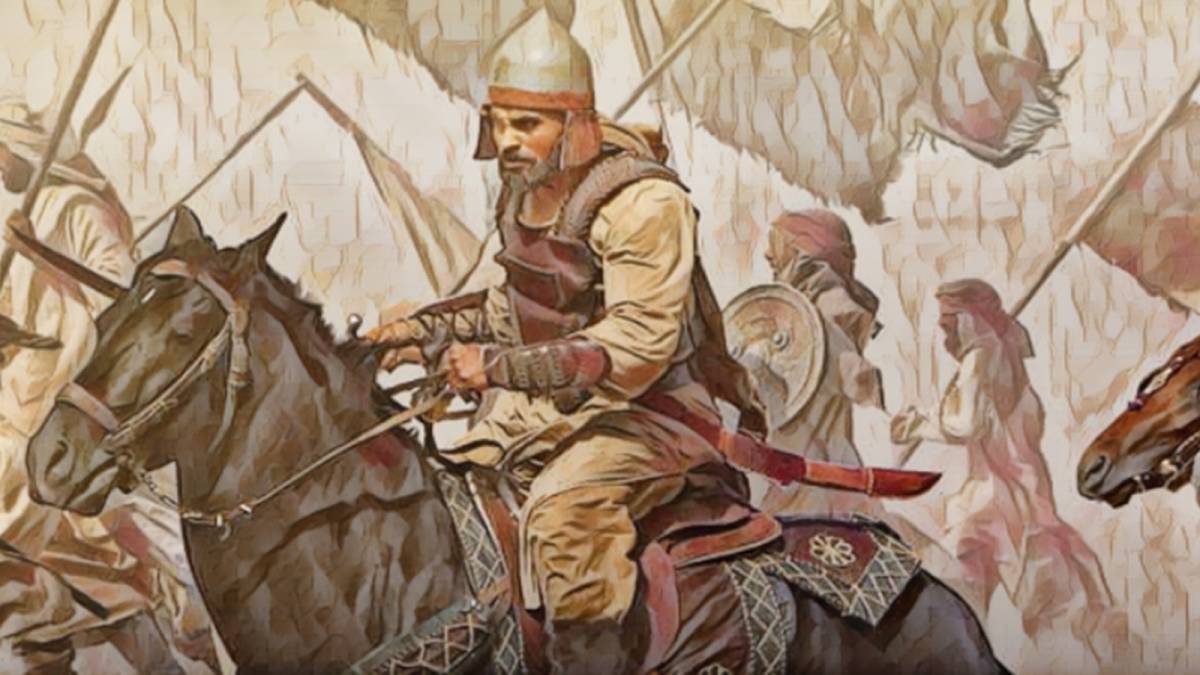The image is a horizontally aligned rectangular painting depicting a fierce-looking warrior from an ancient era, likely the Spartan or Roman Empire. This warrior, who wears a distinctive helmet with a silver and brownish hue and orange rims, sits atop a dark brown horse with a red and brown patterned saddle blanket. He has a pronounced brown mustache and beard, and is attired in a brown vest over tan sleeves and tan pants. The warrior, facing the left side, is the primary focus of the image.

In the background, there are outlines of additional figures, including men carrying spears and one woman holding a flag. The scene suggests a group heading into battle, unified in their direction and purpose. The overall color palette of the background is dominated by brown tones, enhancing the ancient and austere atmosphere of the painting.